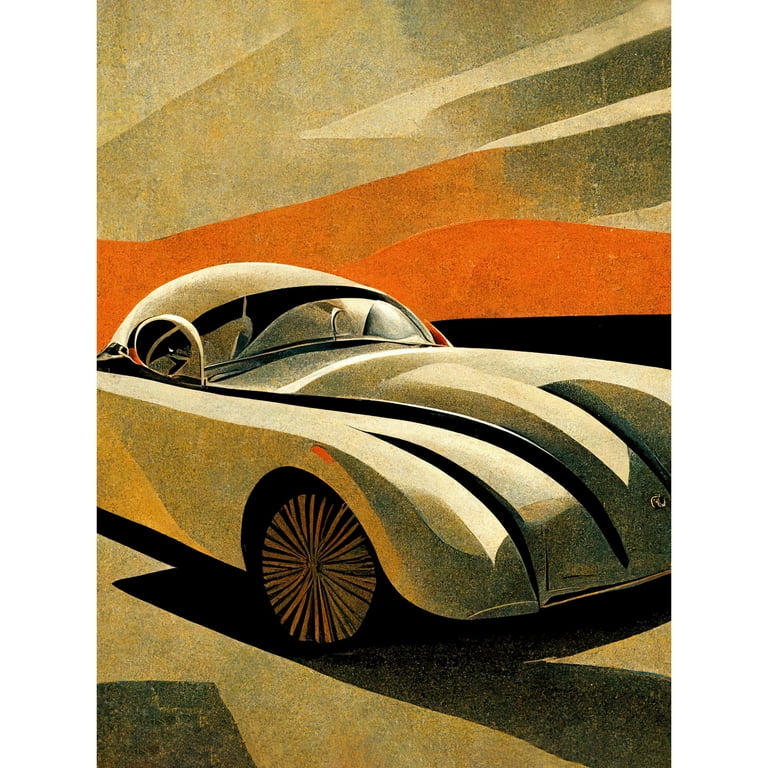This meticulous painting showcases an old-fashioned car in a light yellow and gray color palette. Positioned in a portrait-oriented rectangular frame, the vehicle faces toward the right and slightly downward. The background features an abstract composition of shapes in hues of orange, light gray, yellow, and brown, creating a visually stimulating contrast. A dark gray shadow beneath and to the right of the car adds depth and dimension to the artwork, enhancing its vintage charm.